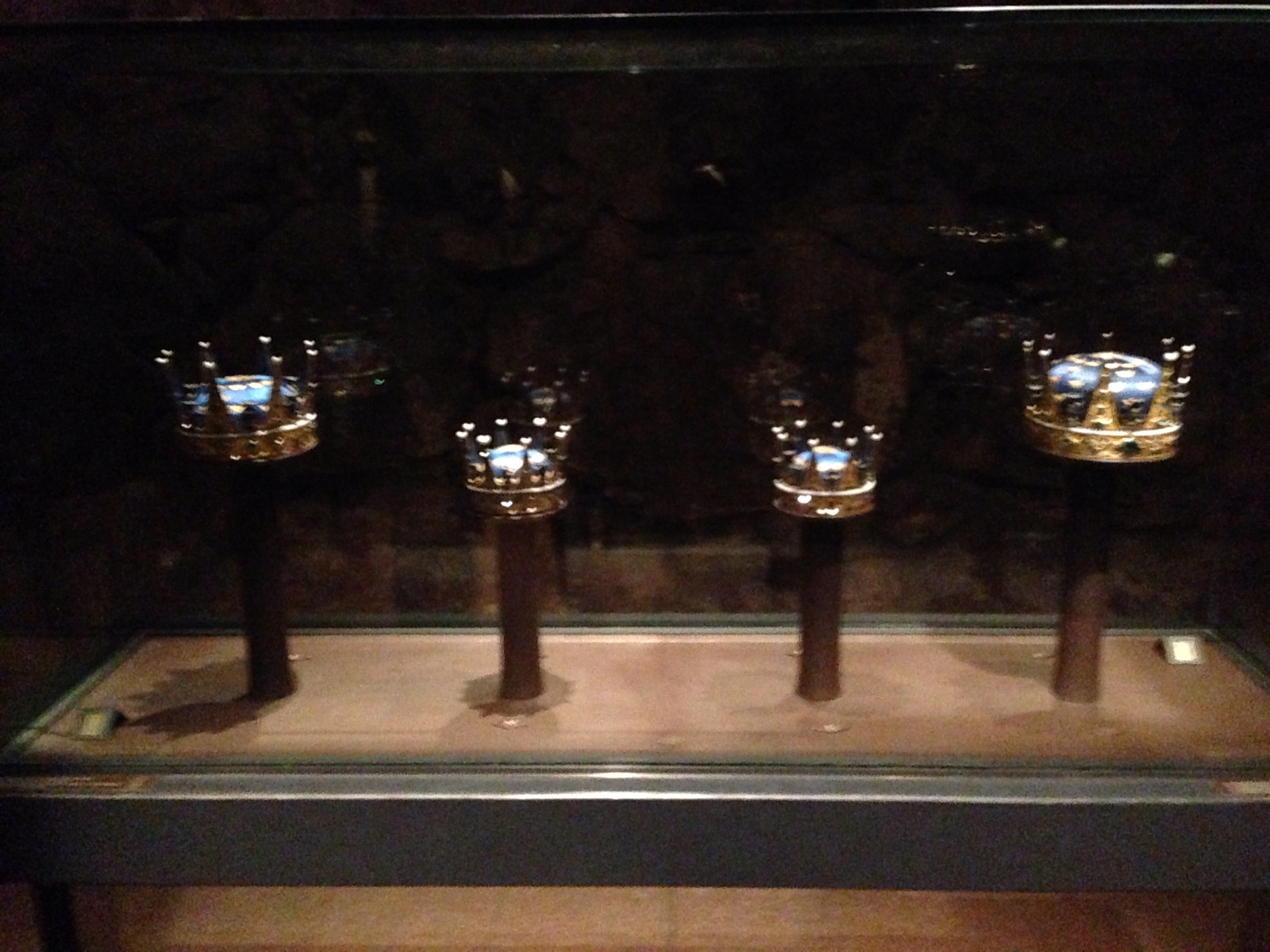The image is a low-quality, blurred color photograph depicting a museum display featuring four crowns, typically worn by royalty such as princes, princesses, kings, or queens. Despite its blurriness, several details are discernible. Central to the image is a table with a light brown wooden surface and a dark grey circumferential surround, possibly enclosed in glass given the visible reflections at the top half of the image. Each crown is mounted on a dark brown metal pole at varying heights, showcasing their different circumferences. The two crowns on the left and right are slightly wider than those in the center. All crowns appear golden with encrusted jewels and traditional peaks around their circumference, accentuated by the museum's focused, low lighting. Additionally, some crowns feature a secondary blue color, potentially fabric. Placards or name tags are visible within the display, which rests on a wooden floor, further framed by a metal boundary, enhancing the regal presentation.